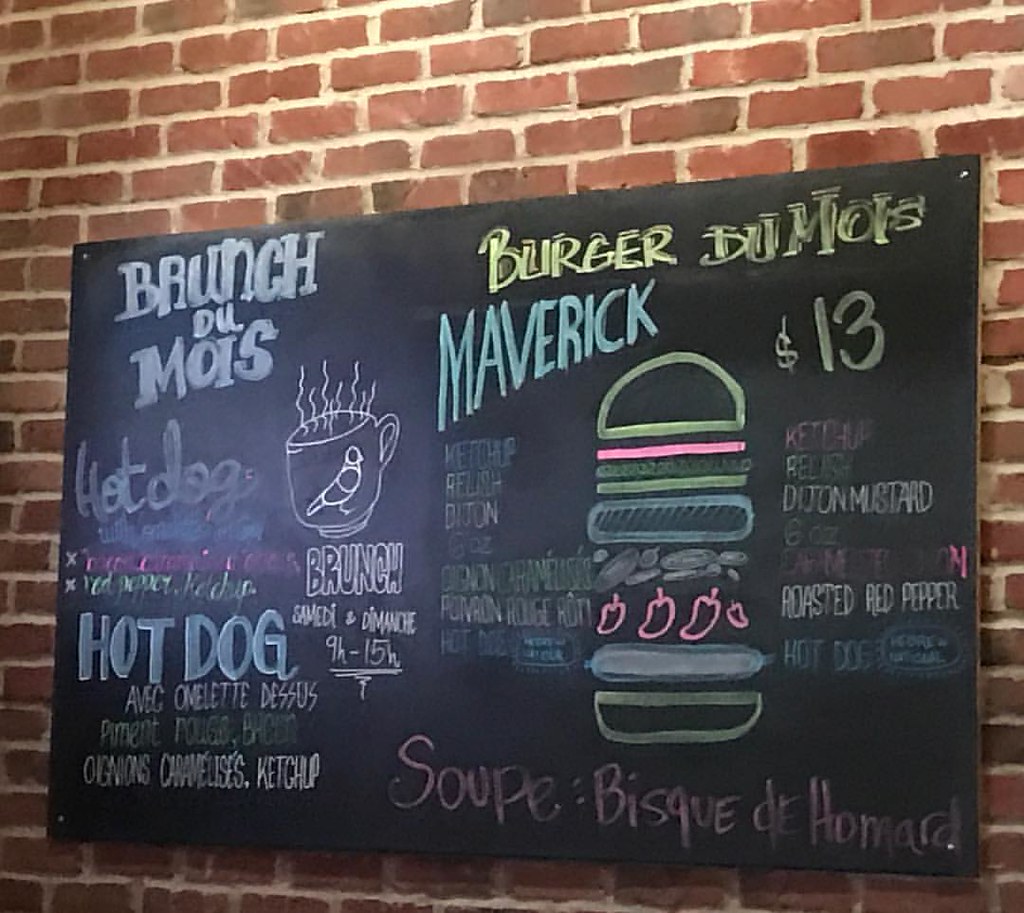The image features a rustic brick wall serving as the backdrop for a chalkboard filled with various colorful drawings and writings. At the top left corner of the chalkboard, the word "Brunch" is prominently written, possibly indicating the name of the establishment, "DuMois." To the top right, "Blues Burger" is noted, also associated with the name "DuMois." 

On the right side, moving from top to bottom, the name "Maverick" is written in blue chalk. In the middle left section, there's a depiction of a hot dog. Adjacent to the right, you'll find a drawing of a beer mug and a bird, alongside wavy lines and the word "Brunch" once more. Beneath this, a code or signature "9H215H" is inscribed.

At the bottom left, "Hot Dog" and "Avocado Omelette" are listed as menu items. Moving towards the center-right part of the chalkboard, a detailed illustration of a burger is showcased: it features layers of green lettuce, a pink tomato, and a big blue patty with various fillings like chopped red peppers and sausage, all enclosed in a bun.

On the left side of the burger, there are depictions of various condiments and toppings that can be added. This section includes items such as ketchup and relish. On the right side of the burger illustration, condiments including Dijon mustard and roasted red pepper are listed. Additionally, "Hot Dog" and a soup named "Bisque de Homard" are also mentioned towards the bottom right corner of the chalkboard.

Overall, the chalkboard presents a vibrant and eclectic menu with detailed illustrations and descriptions of various food items available at this likely brunch spot.